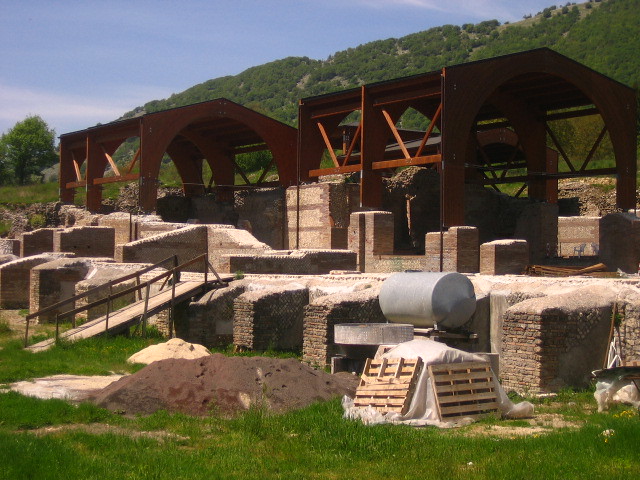The photograph depicts an outdoor scene on a partly cloudy day, framed by a backdrop of lush green hills and trees under a blue sky with wispy white clouds. In the foreground, there is an elevated structure with a base made of light-colored bricks forming a platform that occasionally juts out with shorter brick walls. A wooden ramp, brown with lighter floorboards, ascends to this brick platform. Above the brickwork, there's a canopy or shed-like structure with an arched roof made of rust-colored wood, serving as a cover but lacking walls. Scattered in the grassy area in front of the platform are piles of dark and light-colored dirt, along with pallets holding down a plastic tarp covering an unknown mound. A silverish cylinder lies on its side nearby. The scene has the feel of a building project or an excavation site, with metal foundations or skeletal frames of buildings surrounded by the beginnings of brick walls suggesting construction or preservation activities.